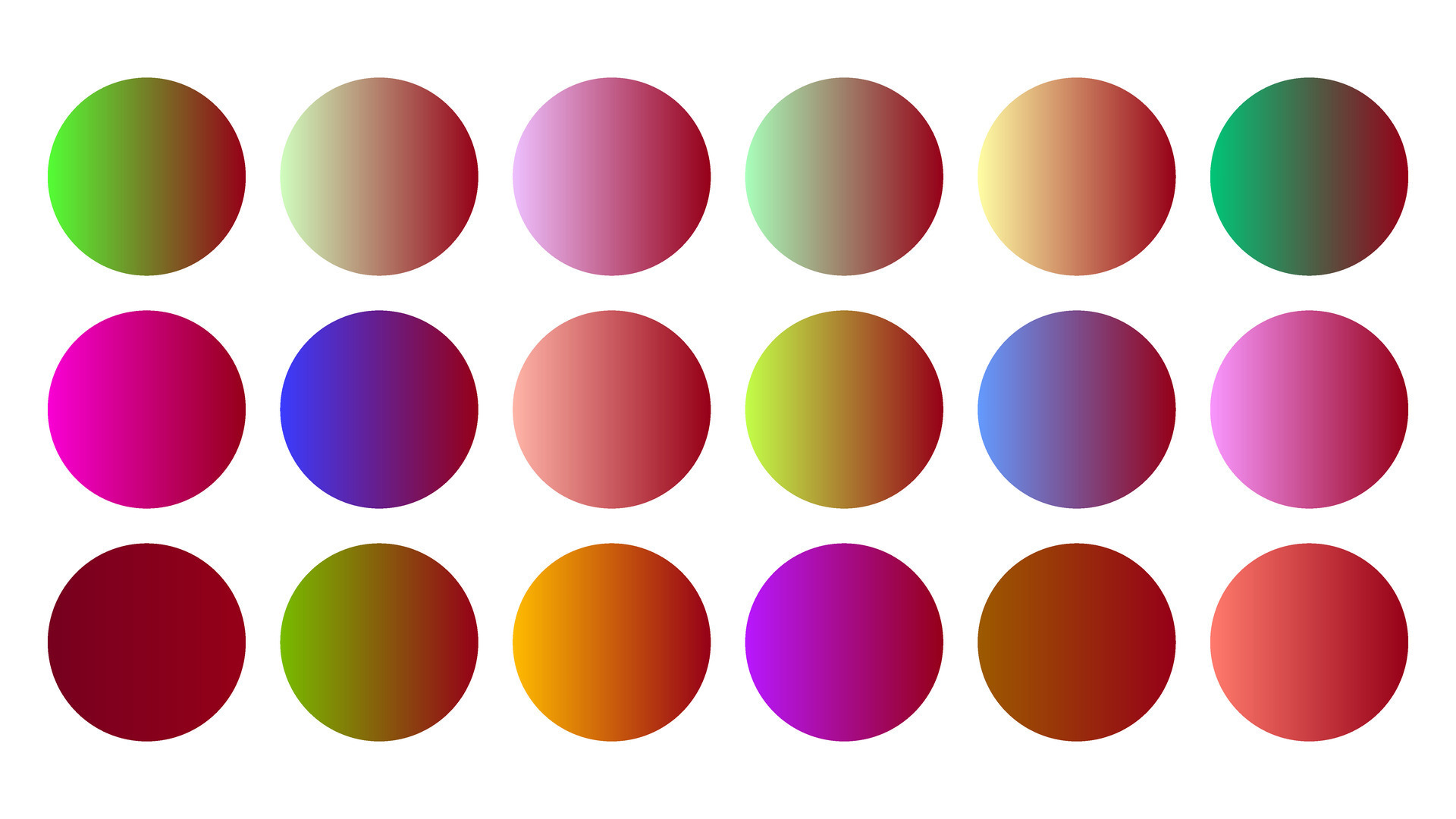This computer-generated image features 18 large, equally sized dots arranged in a grid format on a white background, with six columns and three rows. Each of the vividly colored dots showcases a variety of shades, with some being solid colors while others exhibit smooth gradients transitioning from one hue to another. The first row includes dots in shades like light green, pale green-orange, light purple, green-red, yellow-red, and dark green. Every dot is uniquely colored, featuring a myriad of colors such as purple, green, yellow, blue, orange, maroon, and many variations in between. The overall pattern hints at a blend of colors, possibly showing the transitions and combinations of different hues. The dots are evenly spaced, and the image contains no text or titles to provide additional context.